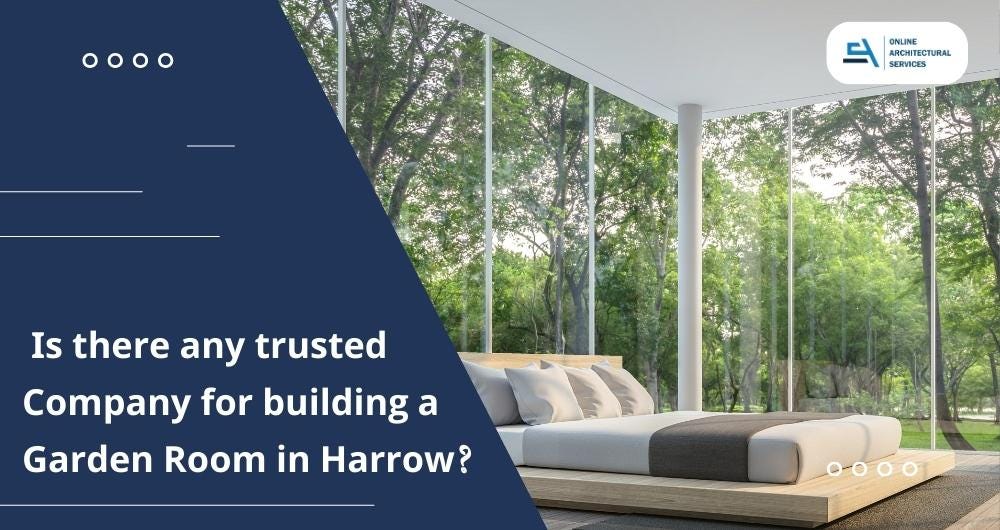The image depicts a screenshot of an advertisement, potentially taken from a PowerPoint presentation, promoting an interior design or architectural service focused on building garden rooms in Harrow. The layout is divided into two sections, with the right section featuring a visually stunning bedroom with floor-to-ceiling glass walls that offer uninterrupted views of a lush, tree-filled backyard. The bedroom contains a minimalist wooden platform bed adorned with four dark tan pillows and layered blankets in shades of gray, brown, and tan, accentuating a modern, futuristic aesthetic. The left section of the image, set against a dark blue background with artistic white lines, displays white sans-serif text asking, "Is there any trusted company for building a garden room in Harrow?" Additionally, a bright teal-colored label in all capital letters at the top right corner reads "ONLINE ARCHITECTURAL SERVICES," emphasizing the digital nature of the advertised services. The image also features interactive white circular buttons for accessing more information, adding a layer of functionality and engagement to the advertisement.